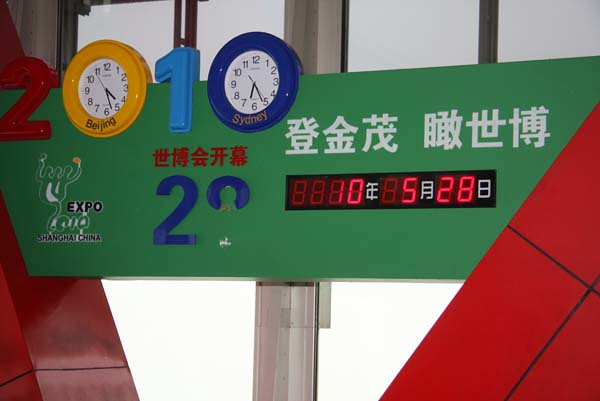The image depicts an indoor scene featuring a highly detailed scoreboard or signboard with several distinctive elements. Dominating the center is a square pole with a long green sign attached to it. Prominently displayed at the top of the sign are three-dimensional numbers that spell out "2010," with each number in a different color: the "2" in red, the first "0" in yellow, the "1" in light blue, and the second "0" in dark blue. The zeros are uniquely designed as clocks; the yellow-cased clock is labeled "Beijing," and the dark blue-cased clock is labeled "Sydney." Below these clocks, there's text that reads "Expo Shanghai China," along with additional Chinese characters. On the lower part of the sign, a large blue number "2" is visible, along with a partial number that appears torn or missing. A digital screen resembling a scoreboard displays the numbers "10," "5," and "28" in red, interspersed with Chinese symbols. The image also includes red structures on either side of the sign, which seem to support it, and glimpses of white walls and possibly daylight filters through in the background, hinting at an exterior view.